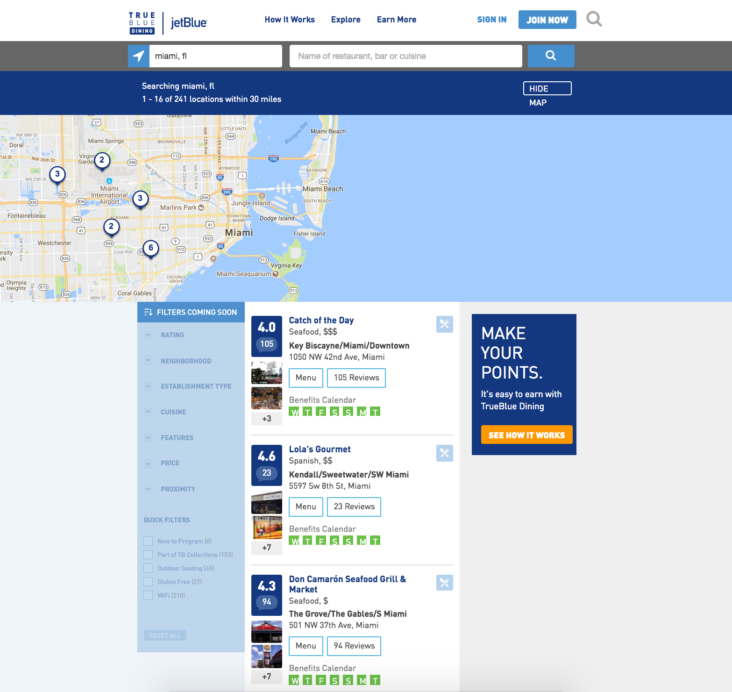The image depicts a webpage from the JetBlue website, showcasing various features and elements aimed at helping users navigate through it. At the top of the page, there are options to 'Sign In' or 'Join Now,' accompanied by a small gray magnifying glass icon to the right. Below these options, there's a search field set to 'Miami, Florida,' indicating the user's location for the search query. Adjacent to this search field, there's another input box labeled 'Name of restaurants, bar or cuisine', designed for users to specify what they are looking for. To the right of this input box, a white magnifying glass icon is set against a blue background, indicating the search button.

Further down, the page displays search results for Miami, Florida, showing 1 to 16 out of 241 locations within a 30-mile radius. Several locations are listed, including Miami Springs, Marlins Park, Coral Gables, Dodge Island, Miami Beach, Miami Seaquarium, and Virginia Key. The interface highlights these destinations, making it easy for users to explore various attractions in and around Miami, Florida.